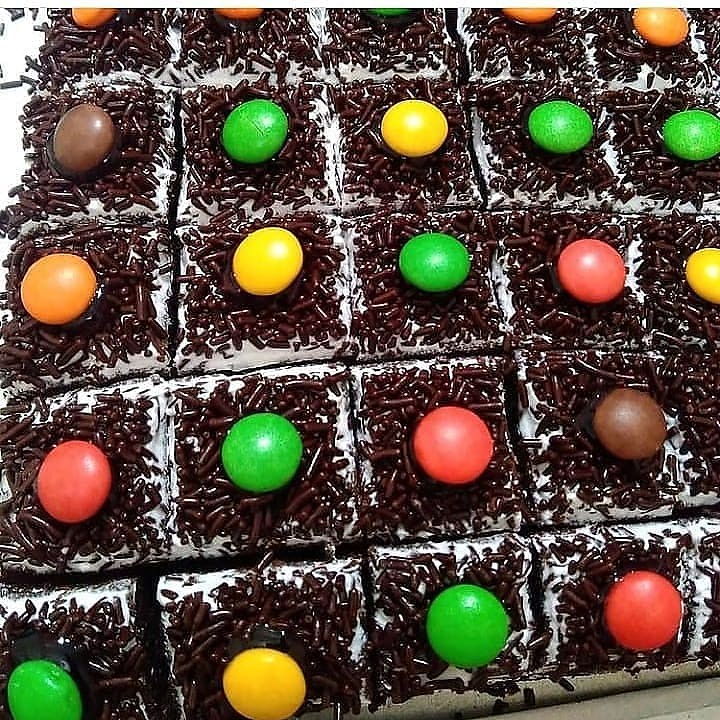This color photograph is a close-up of a chocolate sheet cake or brownie that has been cut into small, roughly one to two-inch square pieces. Each piece of the cake is topped with a layer of white frosting covered in chocolate sprinkles, and adorned in the center with a single M&M candy in alternate colors: green, yellow, red, orange, and light brown. The neatly cut squares, arranged in a grid, suggest there are about 20 to 25 individual pieces visible in the image. The absence of text in the photo highlights the visual appeal of the meticulously decorated treats, possibly home-made and photographed for sharing or sale.